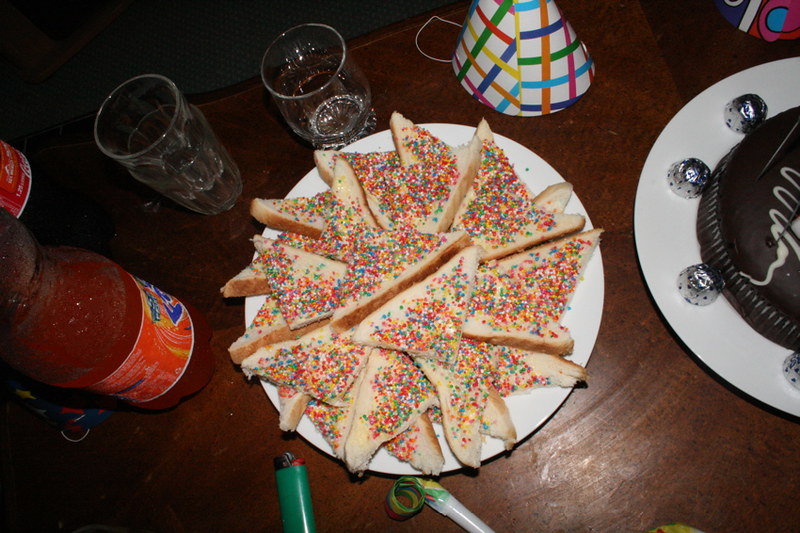This is an overhead color photograph capturing a lively party scene on a dark wooden table. At the center of the image is a white plate stacked with several triangular slices of fairy bread, an Australian treat made by spreading butter on bread and topping it with colorful rainbow sprinkles. Above the fairy bread, slightly to the right, there are two clear shot glasses nested inside each other, with a small clear drinking glass nearby. Directly above the plate of bread sits a festive party hat, adorned with vibrant red, blue, green, orange, and pink diagonal stripes.

To the left of the fairy bread plate, there's a bottle of orange Fanta, which is identifiable by its distinctive orange ring label. Just peeking in from the right edge of the image, about two inches from the top, is the bottom part of a Coca-Cola bottle with a red label. Below the central plate of bread and slightly to the left, a green disposable lighter with a red button on top can be seen. Beside it lies a green noisemaker with a white tip.

To the right of the fairy bread, a white plate partially enters the frame, holding a dark chocolate cake adorned with a white squiggle. Surrounding this plate, four small candies wrapped in aluminum foil are scattered. The table is adorned with an assortment of party items, emphasizing the festive and celebratory atmosphere of the scene.